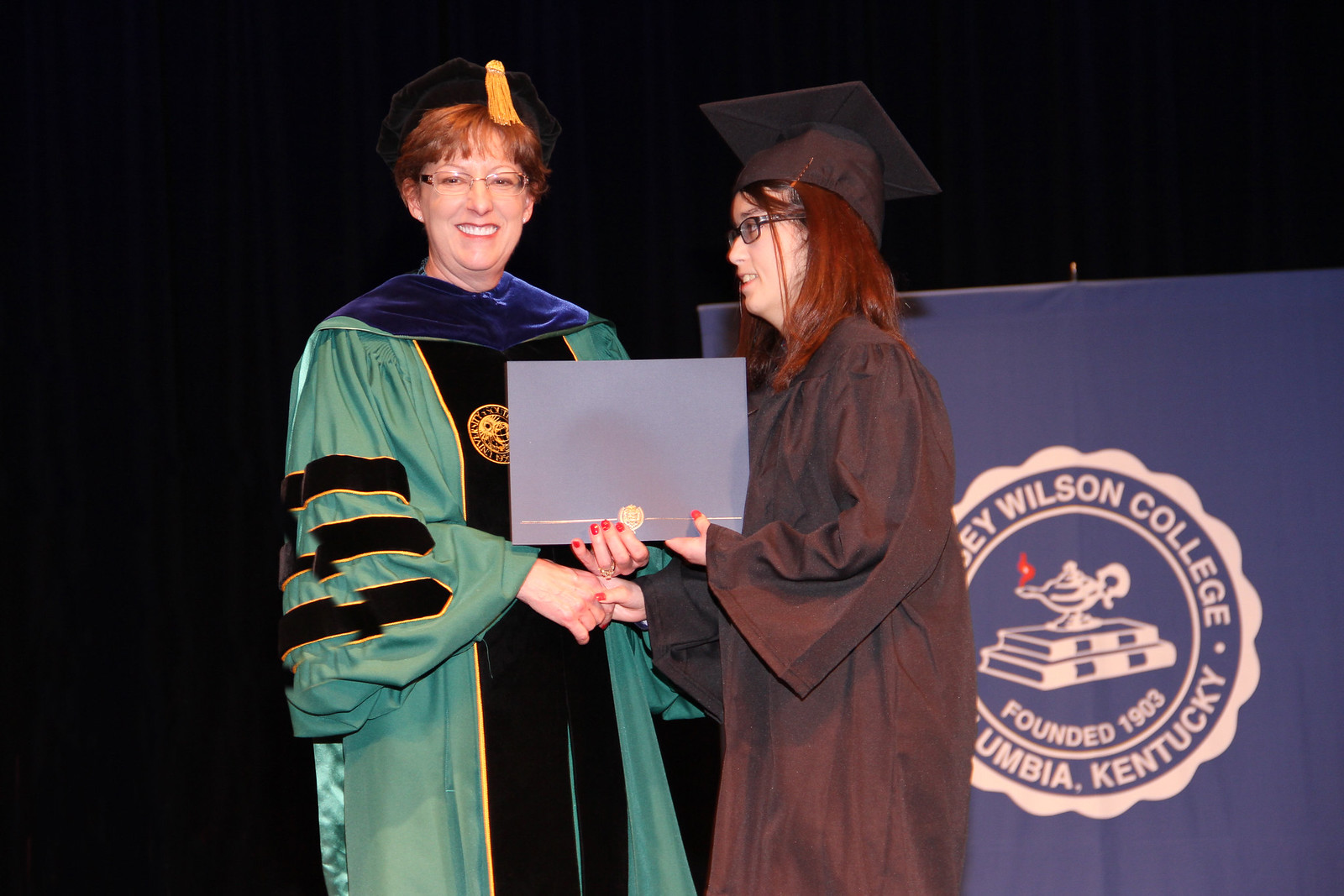In this photograph of a graduation ceremony, a student in a black graduation robe and cap is receiving a diploma from a faculty member. Both are smiling as they hold the blue diploma cover between them, which features a gold line across the bottom. The student, positioned on the right, has long red hair flowing from under her black cap, black glasses, light skin, and pink fingernail polish. She is looking slightly to the left, her teeth visible in a subtle smile. The faculty member, on the left, has short red hair under a black hat with a gold tassel, and also wears glasses. She is dressed in an elaborate robe with royal blue on top, black stripes down the front, light green on the outer sections, and gold and black streaks around the elbows. The background is dark black, and in the bottom right corner, a fabric advertisement partially visible reads "Wilson College in Columbia, Kentucky." It also shows the emblem of two books topped with a mantle and flame, and the words "Founded 1903."